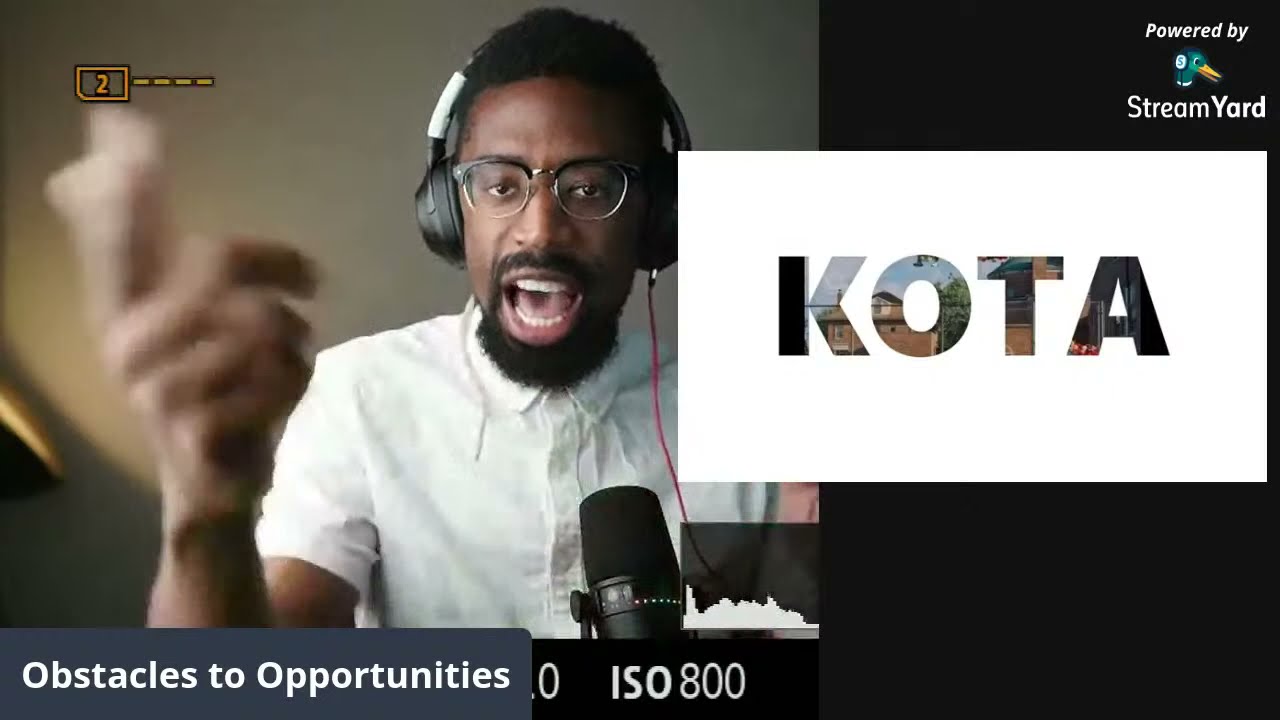The image captures a focused moment of a podcast recording session. Central to the composition is an African-American man, likely in his late 20s to early 30s, with short black hair, glasses, and a distinct black goatee. He sports black over-the-ear headphones with a noticeable white spot on the left side, and is dressed in a white short-sleeve button-up shirt without a tie. Positioned in front of a black microphone, he is speaking passionately, and his raised hand, pointing a finger, appears blurred in motion, emphasizing his dynamic engagement.

The background of the image is split, with the left side featuring a tan color and the right predominantly black. Prominently displayed in the upper left corner is the inscription “Powered by StreamYard” along with an icon of a duck wearing headphones. The lower left corner of the image showcases a gray box with white text that reads, “Obstacles to Opportunities.” Another feature is a large white box slightly intruding from the right, with the letters “K-O-T-A” filled with a cityscape scene, providing a contrast against the dark background. Additionally, a black box beside it displays "ISO 800" in white lettering. This carefully orchestrated visual captures the essence of a modern podcast setup.